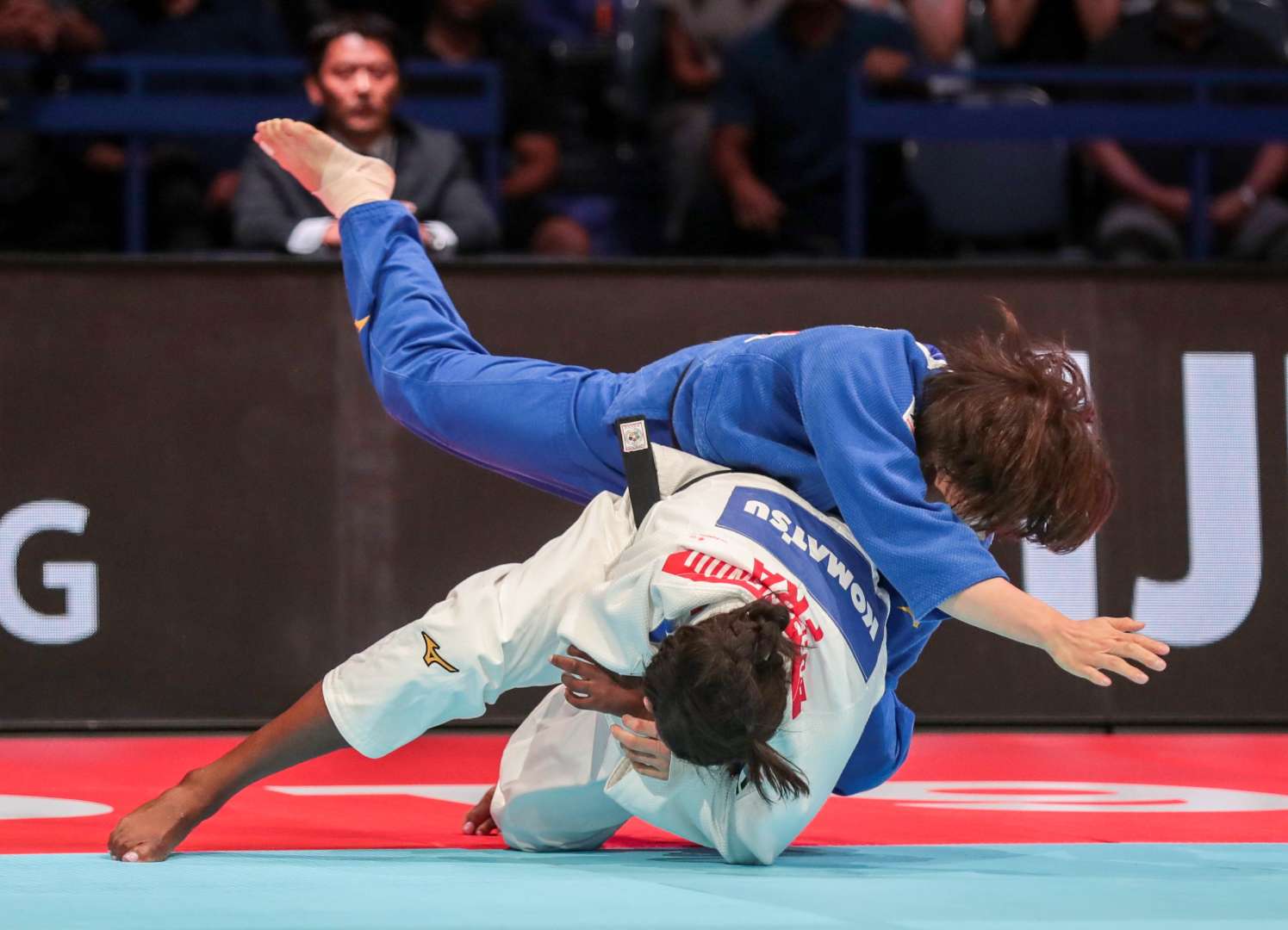This color photograph captures an intense moment in a martial arts competition, likely judo, featuring two barefoot competitors. The athlete in a white uniform, which bears a logo that reads "Komatsu" on his back, lies face down with his right leg outstretched, while the opponent in a blue uniform is positioned on top of him, his right foot extended upward. Both competitors appear to be of differing skin tones; the one in white has brown skin, and the one in blue appears lighter-skinned. The scene is set on an aqua and red mat, which has some unreadable text and is bordered by a black retaining wall adorned with white lettering. The background is somewhat blurred, revealing a crowd of onlookers and blue stands, with an Asian man in a black suit jacket standing near the upper left corner.